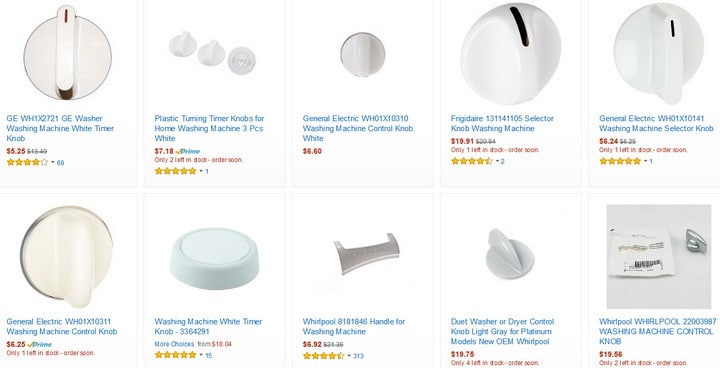Screenshot of a website page dedicated to a shopping site primarily featuring plastic timer knobs. The layout is horizontal, displaying ten timer knobs organized into two rows of five. Each product listing includes an image mainly showing white knobs. Below each image, product details such as the manufacturer's name, a possible model number, and a price in red font along with the full price in black font are displayed. Additionally, a star rating is present under each item, except for the ninth and tenth products on the lower right. Most listings feature single knobs, but the second position on the upper row features a set of three knobs. The third position in the bottom row displays a distinct item, which appears to be a washing machine handle. All images and the website background are predominantly white.